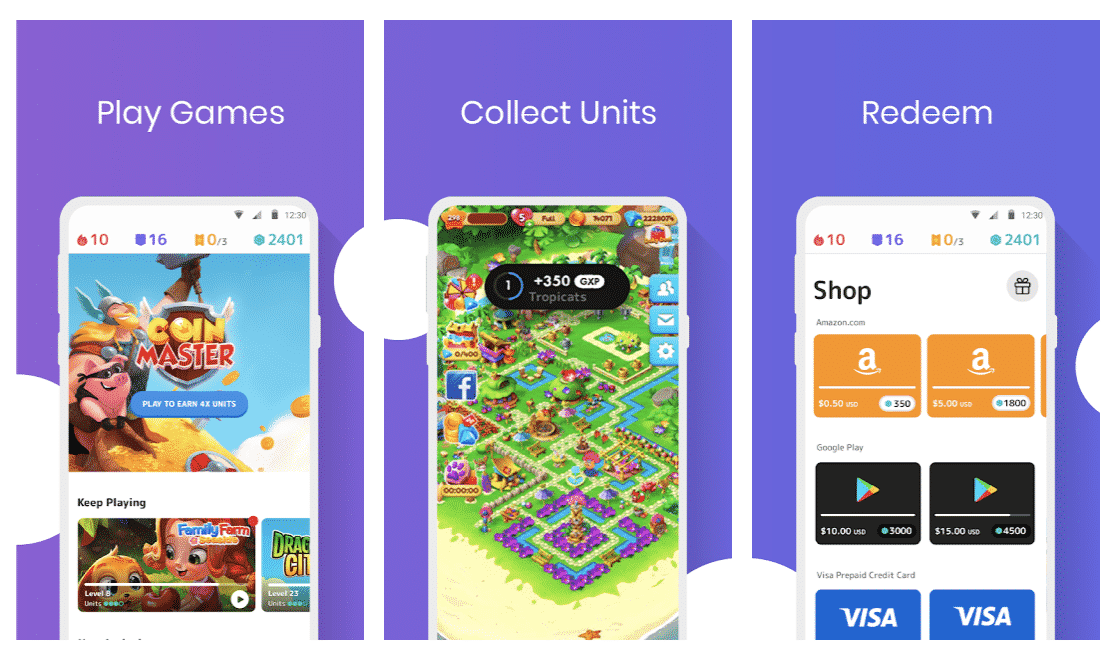The image appears to be a promotional screenshot for a mobile app that rewards users for playing games. The ad is divided into three panels, each set against a purple background and featuring a smartphone with a partially applied layer of sunscreen, perhaps symbolizing the ease of playing anywhere, even by the pool or beach.

1. **Left Panel: "Play Games"**
   - At the top, the text "Play Games" is prominently displayed in white.
   - The smartphone screen shows the mobile game "Coin Master," featuring cartoon characters, including a pig and a person. The game scene suggests dynamic and engaging gameplay.

2. **Middle Panel: "Collect Units"**
   - The heading "Collect Units" appears at the top in white text.
   - The phone screen displays a game with a retro, 8-bit or 16-bit art style, set in a landscape environment. A label reading "+350" appears in an oval, indicating points or units collected.

3. **Right Panel: "Redeem"**
   - The top of this panel features the word "Redeem" in white text.
   - The phone screen shows a shopping interface with the word "Shop" in black text.
   - There are visuals of gift cards from Amazon, Google Play, and Visa, suggesting that users can redeem their collected points for these rewards. Some logos are partially cut off, but the intent remains clear.

Overall, this ad promotes an app where users can play different mobile games, accumulate points, and redeem those points for various gift cards.